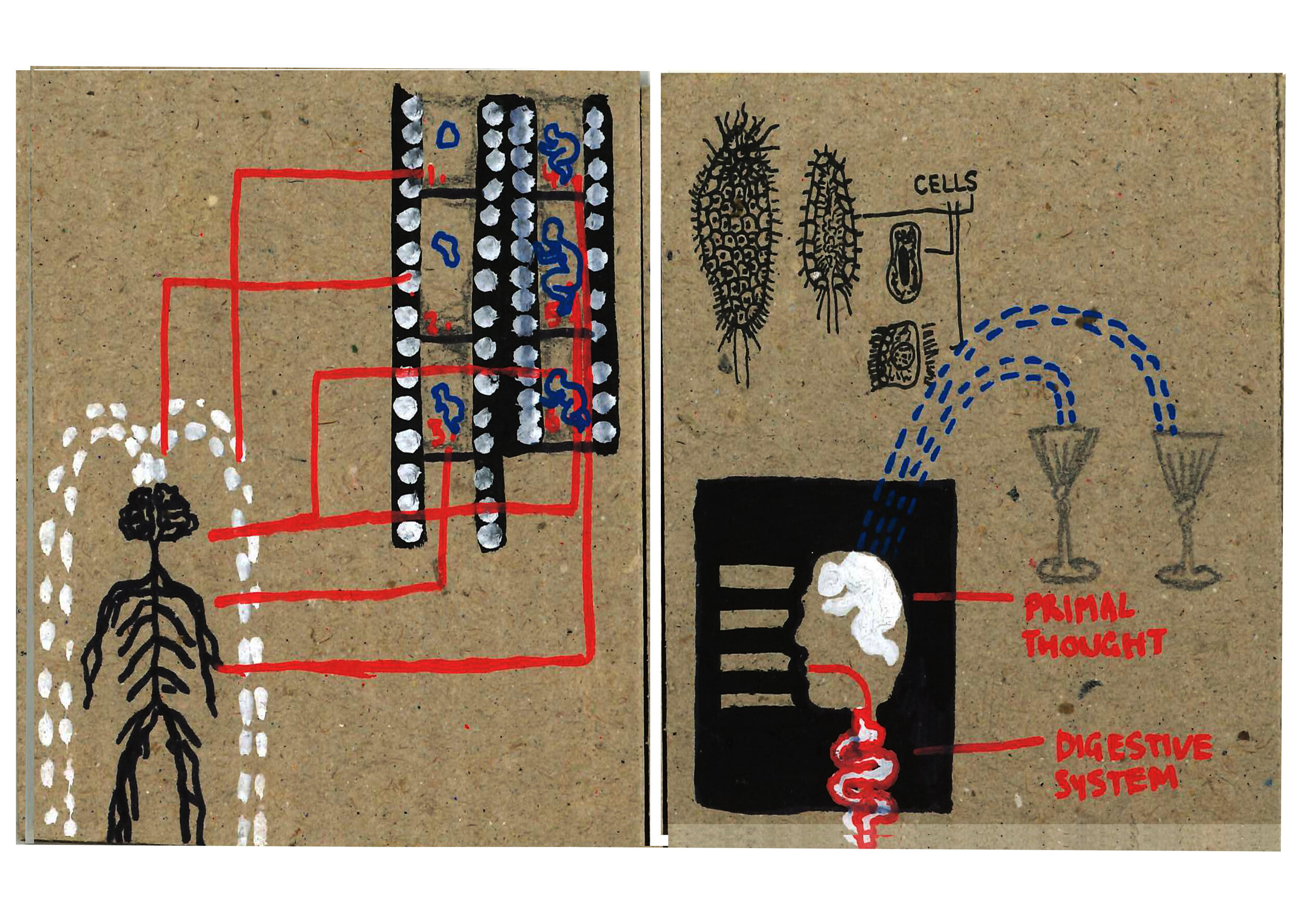The artwork, crafted on cardboard canvases, features two distinct yet thematically connected hand-painted illustrations. The left side depicts a skeletal human figure with exposed ribs, seemingly weeping profusely with white dots streaming from its eyes, reminiscent of a waterfall. These droplets then get funneled into what appears to be a wine cellar. Capping the figure's head is a striking white fountain, bordered by emanating red lines. The illustration on the right presents a scientific diagram-like scene with two glasses of water pouring liquid into a human head, complemented by labels such as "primal thought" and "digestive system" written in red letters. This conceptual piece blends anatomical and metaphorical elements into a poignant visual narrative.